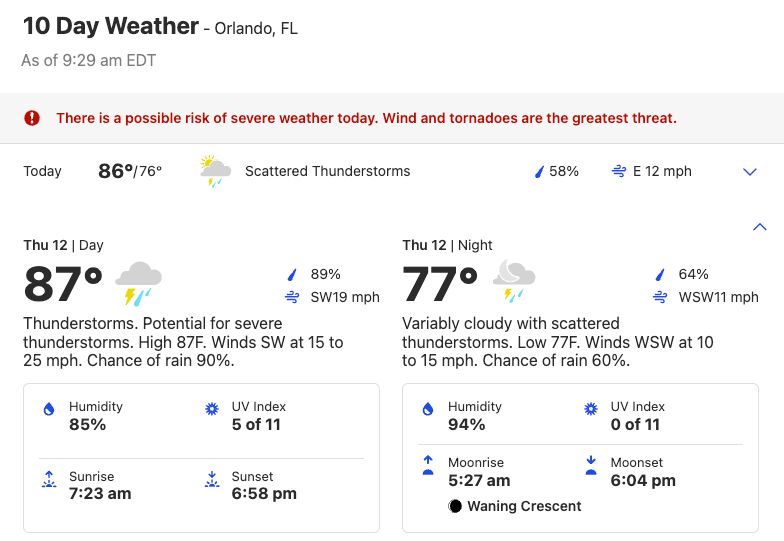The screenshot displays a detailed 10-day weather forecast for Orlando, Florida, with information as of 9:29 a.m. EDT. In the upper left corner, it states "10-day weather - Orlando, Florida." Just below this, in a smaller gray font, it confirms the current time of the report. A notable gray banner with a red exclamation mark inside a circle warns: "There is a possible risk of severe weather today. Wind and tornadoes are the greatest threat."

In the forecast section, the current day's weather is highlighted:
- **Date:** Today
- **Temperature:** 86°F / 76°F
- **Weather Icon:** A sun partially obscured by a cloud, with raindrops, representing scattered thunderstorms
- **Rain Probability:** Indicated by a raindrop icon and 58%
- **Wind:** East at 12 miles per hour

The forecast also extends to Thursday, the 12th of the month:
- **Daytime (Thursday 12th):**
  - **Temperature:** 87°F
  - **Weather Icon:** A cloud with lightning bolts and raindrops, signaling thunderstorms
  - **Rain Probability:** Not explicitly mentioned in this part
  - **Wind:** Southwest at 19 miles per hour
- **Nighttime (Thursday 12th):**
  - **Temperature:** 77°F
  - **Weather Icon:** A cloud with a moon and raindrops, indicating nighttime rain
  - **Rain Probability:** 64%
  - **Wind:** 11 miles per hour

Additional details below the temperature metrics cover aspects like humidity, UV index, and sunrise/sunset times, ensuring a comprehensive weather overview for the upcoming days.